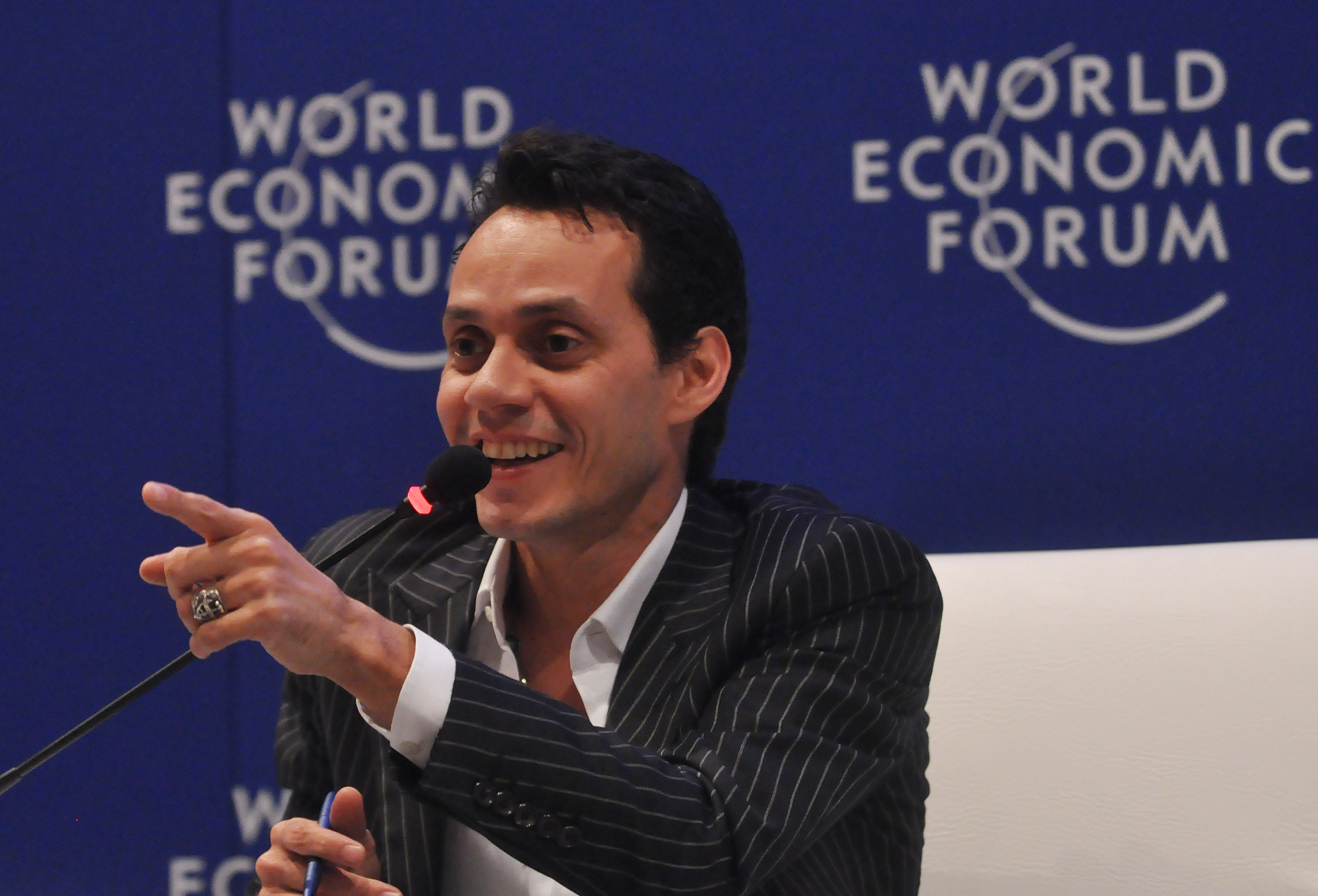The photograph captures the famous Puerto Rican singer Marc Anthony as the central figure. He appears to be speaking into a black microphone with a distinctive red band. Marc Anthony is smiling and gesturing with his left hand, pointing towards the left side of the image. He is attired in a stylish, dark grey overcoat jacket adorned with white pinstripes, under which he wears a white collared shirt. The overcoat features five black buttons. In his right hand, he holds a blue pen. The background showcases a blue banner with the white, uppercase text "WORLD ECONOMIC FORUM" alongside a half-circle design. A white strip or section occupies the bottom right of the backdrop. Marc Anthony's short, dark hair and clean-shaven face are clearly visible, making him the unmistakable focal point of the image.